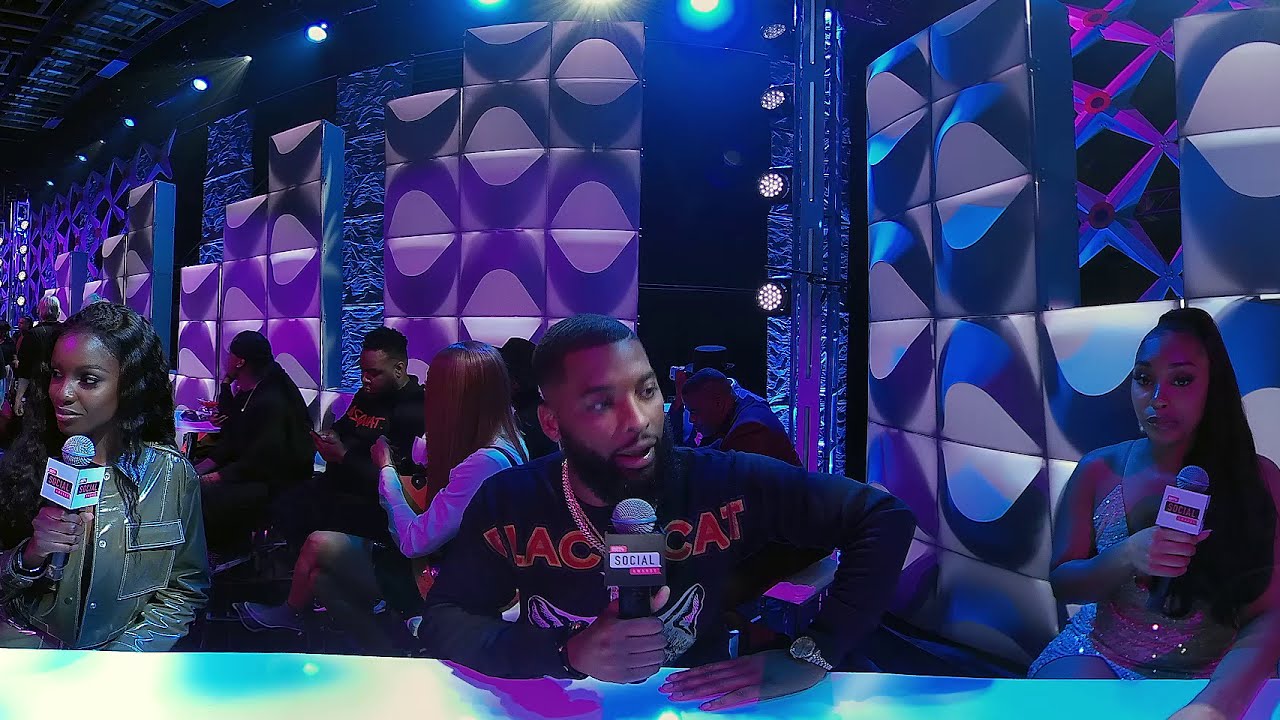In this horizontal, rectangular image, a trio of announcers appears to be on a stage set or monitoring an event. The setting is a dark interior, potentially a nightclub or an evening sporting event, filled with a busy array of purple shapes, circles, and lights that illuminate the background from behind and above. Central in the foreground is a black man holding a microphone, wearing a shirt emblazoned with "Black Cat" and a gold chain, seemingly speaking as he leans on a table or counter. Flanking him are two women, each also holding microphones bearing their network's branding. The woman on the left, visible in greater clarity, appears to be momentarily silent, while the woman on the right might be in the middle of talking or poised to start. The dynamic lighting and the focused expressions suggest a lively commentary scene.